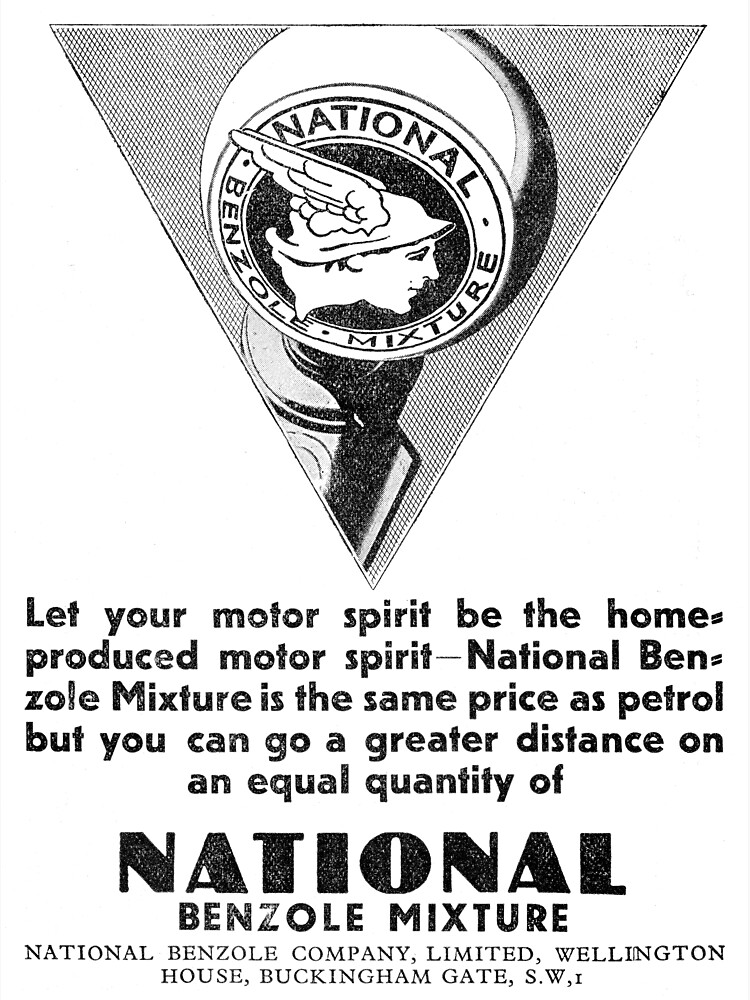This grayscale magazine advertisement for National Benzel Mixture features a prominent downward-facing triangle with a mesh-bordered logo at the top. Within the triangle is a circular emblem displaying the text "National Benzel Mixture," encircled by a sphere that resembles a gas pump handle. The centerpiece graphic, reminiscent of the FTD florist character, depicts a man's face adorned with a helmet that has wings extending from it. Beneath this design, a cylinder-like element extends downward. The advertisement's text reads: "Let your motor spirit be the home-produced motor spirit. National Benzel Mixture is the same price as petrol but you can go a greater distance on an equal quantity of National Benzel Mixture." The bottom of the ad provides the company details: "National Benzel Company Limited, Wellington House, Buckingham Gate, S.W.1."